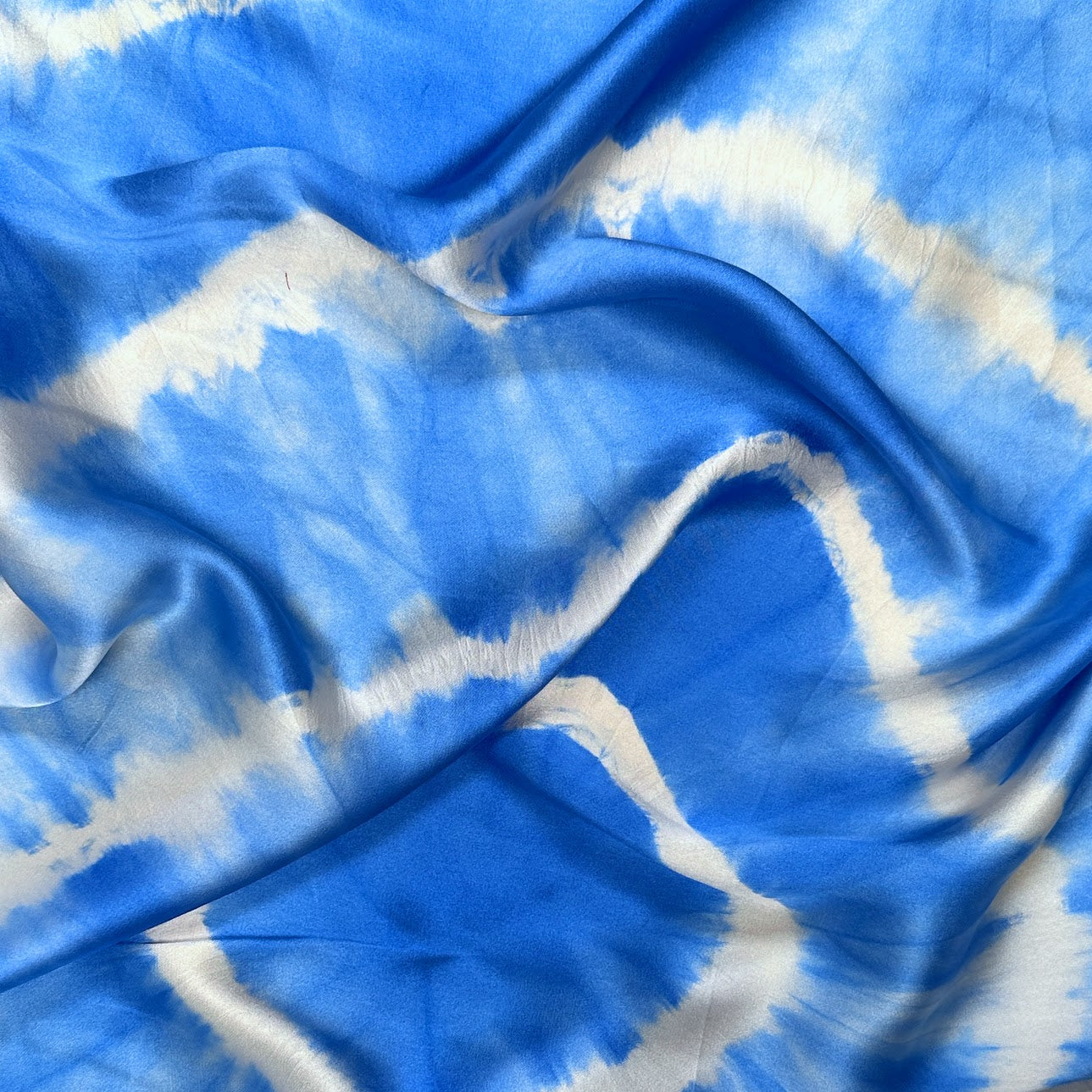This extreme close-up photograph captures a blue and white fabric, intricately showcasing a mesmerizing tie-dye design. The fabric appears to be slightly ruffled, sporting large wrinkles particularly towards the top, bottom left, and bottom right. While most of the surface is uneven, some sections lie relatively flat, revealing subtle patterns that might be part of the fabric’s print or due to the creases themselves. Predominantly blue, the fabric features wisps of white that converge to form concentric circles with varying intensities of color. A darker central circle is most prominent, starting from the bottom middle left, with lighter bands radiating outwards and appearing more pronounced towards the upper left. The fabric’s random folds and wrinkles add a dynamic texture, drawing attention to the captivating, almost sky-like pattern. The lower right corner seems to have more white, though this could be an effect of the fabric’s folds. The tight framing of the photo focuses solely on the fabric, leaving no clues about the surrounding environment.